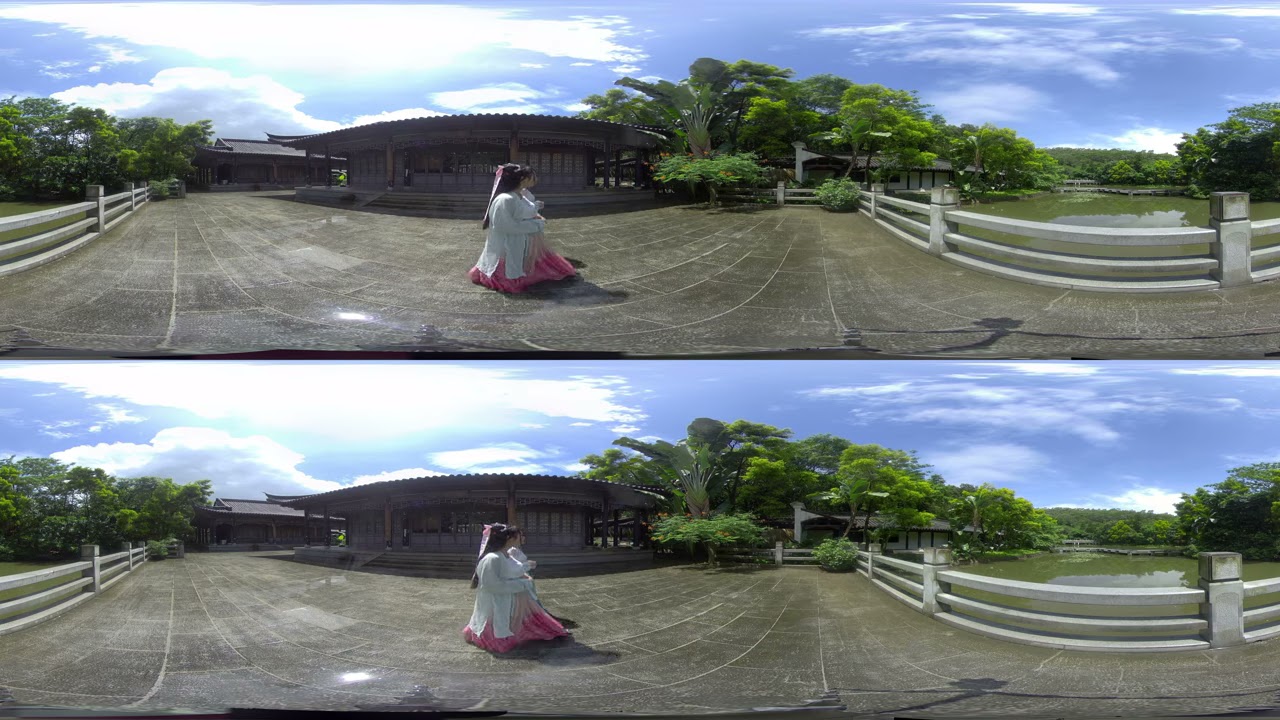In this duplicated photo scene, a young woman stands in the foreground, dressed in a knee-length purple-pink dress and a flowing white cardigan. Her long black hair, adorned with a pink bow, cascades freely down her back as she looks away from the camera. The image captures her in the driveway of a traditional Japanese-style wooden home, surrounded by lush greenery. On the right-hand side, there is a serene green pond bordered by a white fence, nestled amongst bamboo and other Japanese trees. The scene unfolds under a bright blue sky with a few clouds, though the upper left corner is slightly overexposed, giving it an ultra-white glow. In essence, the two vertically stacked identical images evoke a tranquil, picturesque setting, highlighting the harmony between the built and natural elements.